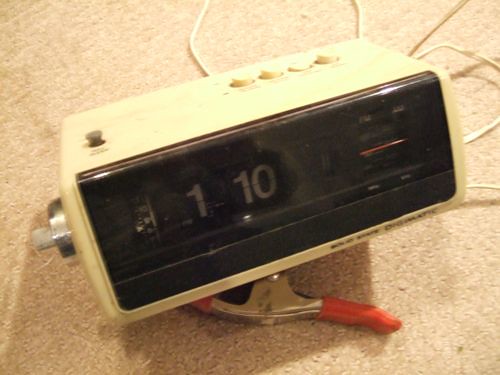In this image, we see a vintage alarm clock with a rotary-style display system. The clock face features a black background with white numbering, showing '1' on the left and '10' on the right, indicating a mechanical mechanism that rotates to display the changing time, rather than a digital readout. On the right side of the clock, there is a red line adjacent to a tuning dial, suggesting that this device doubles as a clock radio. The word "Digimatic" is printed at the bottom of the clock face.

The alarm clock's casing is a vibrant yellow, and it is equipped with four yellow buttons and one gray button on the top, though the labels for these buttons are not visible. The clock is placed on a tan-colored carpet. Additionally, near the clock, there's a piece of silver hardware with a red rubber tip, though its exact purpose is unclear from the image.